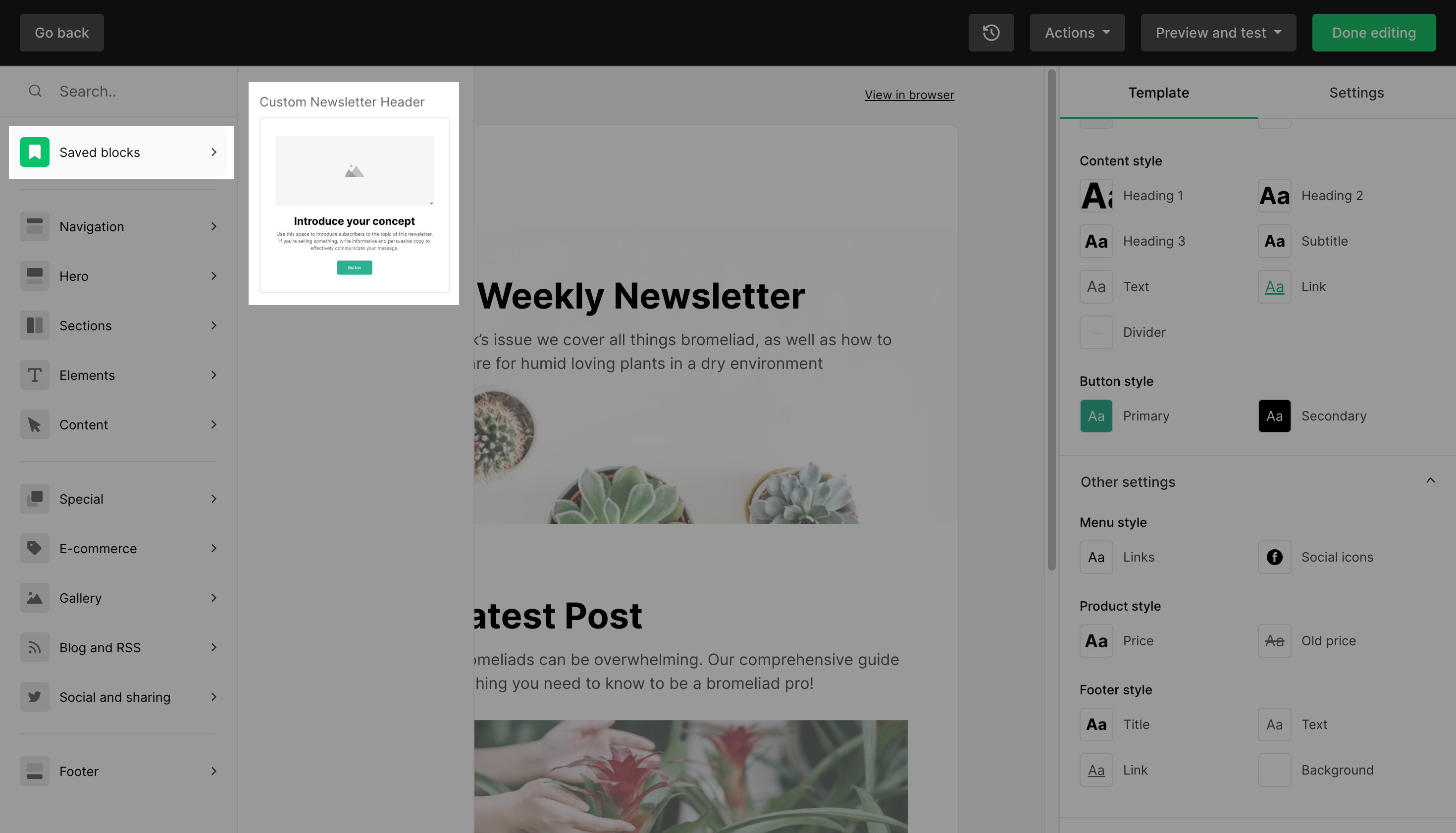The image is a screenshot from a website that appears to be in an editing mode, as indicated by various highlighted sections and buttons. The overall appearance of the webpage is slightly grayed out, except for specific highlighted areas. 

At the top of the image, the background is entirely black. Positioned in the top left corner is a rectangular button with the text "Go Back" displayed inside it. On the top right corner, there is another button with a green background stating "Done Editing."

The main part of the webpage, which is usually white, appears grayed out in the image. However, two particular sections stand out in white. One section is labeled "Saved Books" with an arrow pointing to the right. The other highlighted white section contains the text "Custom Newsletter Header," accompanied by some additional writing.

In the center of the image, there is a segment titled "Weekly Newsletter" that includes a picture of plants underneath the heading. Below this, there is another section intended to display the text "Latest Post," though some of the letters are cut off. Directly beneath this title, there is an image of hands holding a flower.

Additionally, on both the left and right sides of the page, there are lists of various options that the user can choose from. These lists are presumably part of the webpage's editing tools.